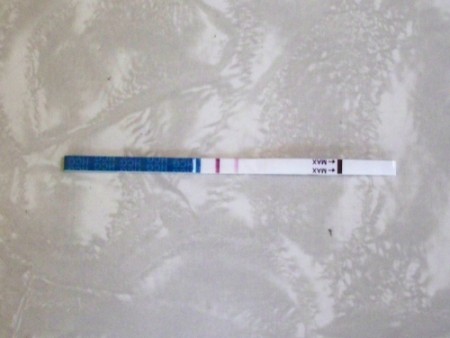This image captures a pregnancy test lying horizontally on a textured, white surface that resembles close-up bubble wrap, with its characteristic bumps and indentations creating a unique backdrop. The pregnancy test stick runs from left to right. The left end of the stick is blue and features the white lettering "HGC" repeated five times around its circumference. Adjacent to this blue section is a thin white band encircling the stick, followed by a blue band, then a white band and a thin red band in sequence. Another white section, more square in shape, leads to another thin white band. Towards the right end of the stick, there's a black band with two arrows pointing towards it and the word "MAX" printed twice upside down, indicating the top of the letters facing the bottom of the image. The stick terminates with a plain white tip extending about an inch beyond the black band.